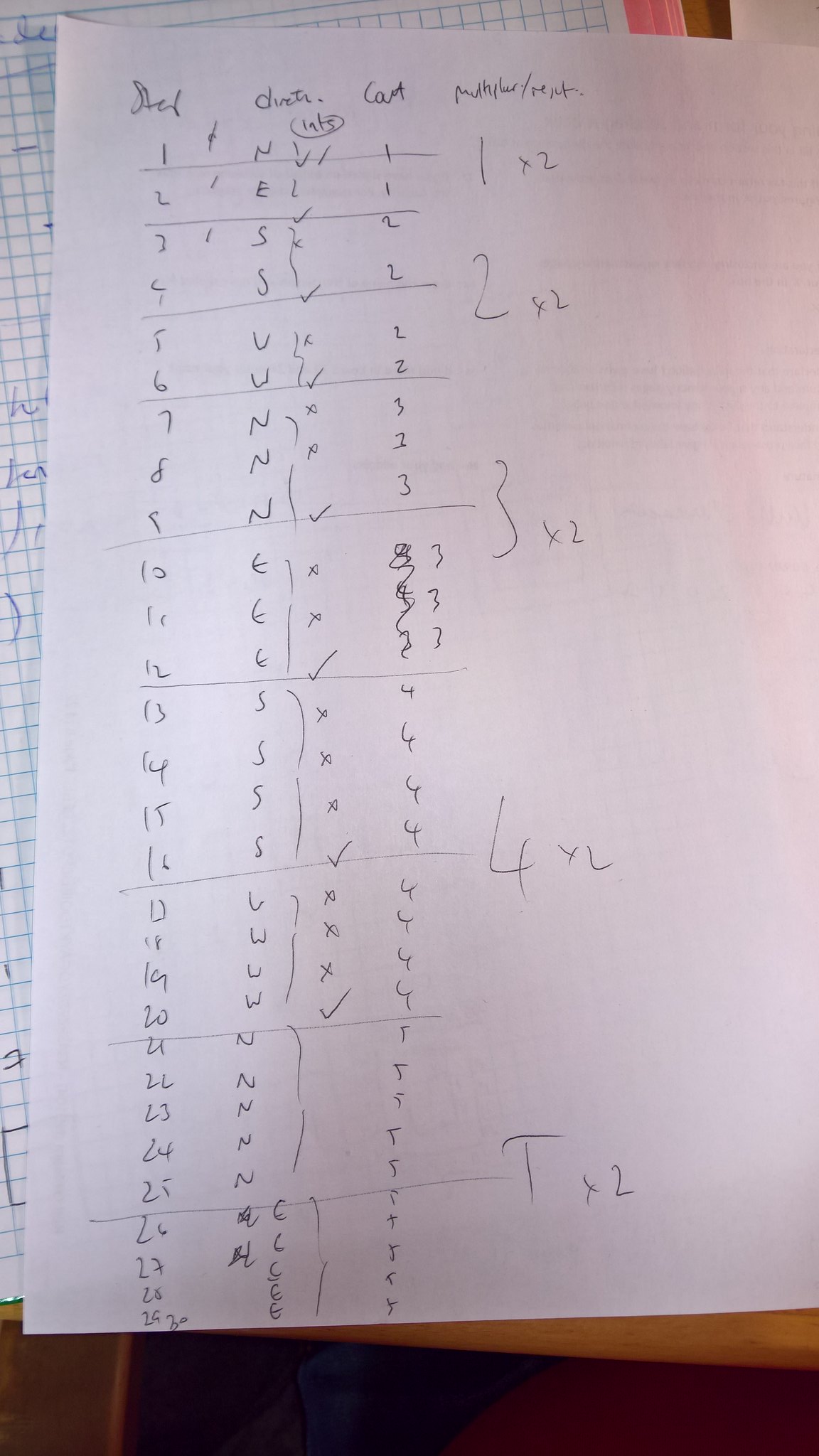A wooden table with a rich, brown finish is adorned with various papers, including a notable large white sheet detailed with numerous numerical calculations, sectioned methodically. Beneath this, a partially visible piece of graph paper, recognized by its small blue grid, also contains handwritten notes. The floor beneath the table shares a wooden texture, complementing the furniture above. The white paper prominently displays multiple sequences of calculations such as "1 x 2," "2 x 2," followed by "3 x 2," "4 x 2," and intriguingly, "T x 2." These numeric sections are interspersed with checkmarks and intersected by lines, signifying methodical segmentation. A closer look reveals some entries have been overwritten, indicating revisions or updates. Though the specific purpose of these numbers remains elusive, it is evident that this document involves detailed tallying or computations.